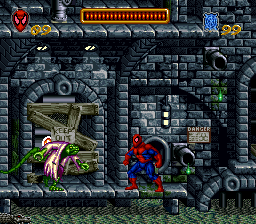The image depicts a scene from a Spider-Man themed video game. In the upper left-hand corner, a Spider-Man mask icon is prominently displayed alongside a fully charged power bar. Additional symbols, likely indicating lives, weapons, or other game mechanics, are seen beside the power bar. The setting features stone walls and a doorway that has been boarded up, suggesting an abandoned or hazardous environment. The lighting is minimal, with just a hint of illumination highlighting the rugged concrete edges of the location. In the center, a creature resembling a blizzard-like being with wings appears, adding an element of imminent peril. Positioned on both the left and right sides of the image, Spider-Man is crouched in a defensive stance, arms flexed as if ready to engage in combat. A sign on the back wall ominously warns of "danger," amplifying the sense of urgency and threat in the scene.